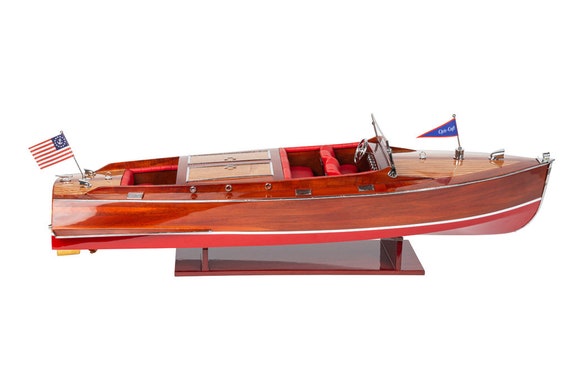The image features a detailed model of a vintage motorboat, poised elegantly on a wooden stand against a stark white background. The boat is primarily made of wood with a luxurious mahogany color, giving it a glossy and waterproof appearance. The bottom and interior seats of the boat are highlighted with a striking red, complimenting the rich brown of the sides. Positioned to the right, the boat showcases its design, reminiscent of a 1960s speedboat, suggesting its history as a precursor to modern ski boats. Two flags adorn the vessel: at the front, a blue triangular flag with a red border and indecipherable white text, and at the rear, an American flag featuring an unusual symbol in the blue canton. Central to the boat, behind the driver's seat, lies a storage compartment with dual doors, lined with red felt-like material, enhancing its vintage charm. The boat's detailed craftsmanship and poised display highlight its classic and timeless appeal.